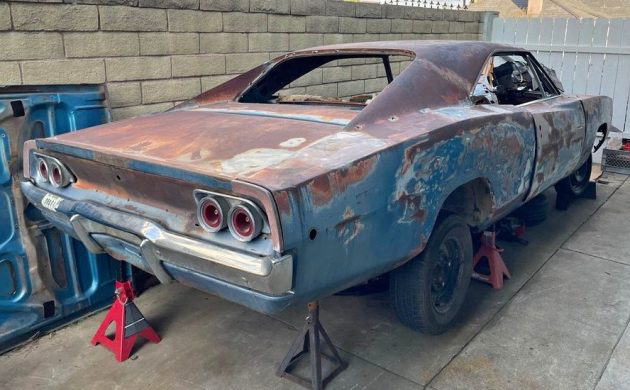The photograph features an old, dilapidated, blue sports car situated outdoors in a driveway, which resembles a sidewalk in texture. The car, originally a medium blue but now heavily rusted on the top with dark brown and gray patches, is held up by multiple jacks, lifting it off the ground to suggest ongoing maintenance or long-term abandonment. The two-door car shows significant signs of wear, including the complete absence of windows. Two visible tires remain attached. The scene reveals the back right corner of the car, where twin red circle taillights and a silver bumper can be seen. Surrounding the driveway is a gray stucco brick wall on one side and a light gray painted fence, possibly a white picket fence, on the other. Additionally, a blue metal appliance is placed between the wall and the car, further indicating the cluttered and neglected condition of the scene.